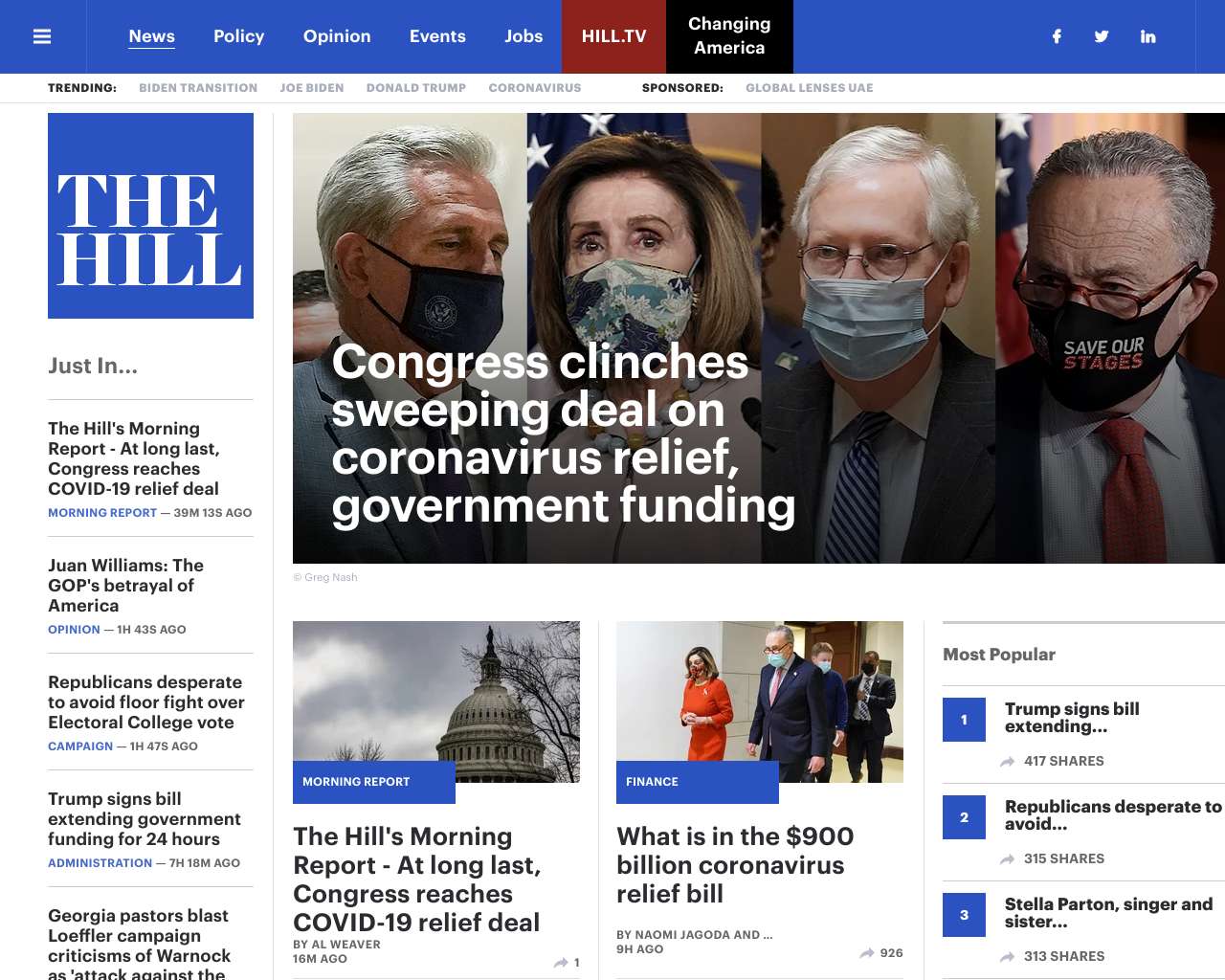The image is a screenshot from the HEAL website featuring a detailed news article. At the top right corner of the image, the headline reads, "Congress Clinches Sweeping Deal on Coronavirus Relief, Government Funding," accompanied by photographs of four government representatives donning face masks. Below this, there's an image capturing the top of the Capitol building, labeled "Morning Report: The Hill's Morning Report - At Long Last, Congress Reaches COVID-19 Relief Deal."

Adjacent to this, on the right side, there's a banner titled "France" and a coverage titled "What is in the $900 Billion Coronavirus Relief Bill?" This segment shows four people walking, all wearing masks. Further to the right, there is a "Most Popular" list which includes three headlines: 1) "Trump Signs Bill Extending," 2) "Republicans Desperate to Avoid," and 3) "Stella Parton, Singer, and Sister."